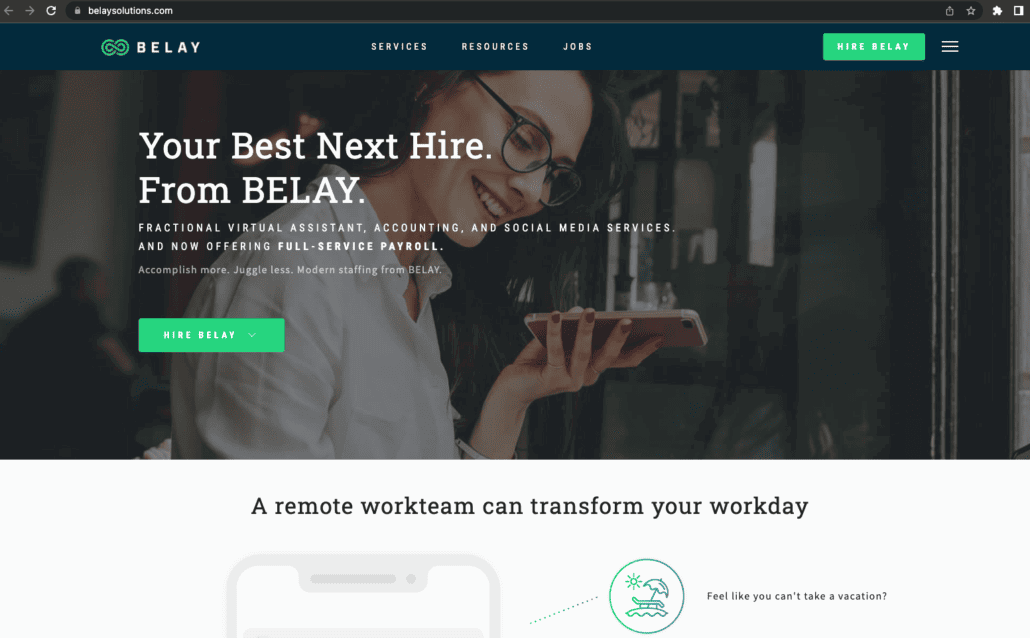The screenshot depicts an advertisement for BeLay, a company specializing in virtual assistance. The BeLay logo, featuring a green infinity symbol to the left of the word "BeLay," is prominently displayed. Running across the top of the advertisement is a black banner with white menu options for "Services," "Resources," and "Jobs." To the far right, there's a green button labeled "Hire BeLay" next to a menu icon consisting of three vertical bars.

Below the banner, a headline reads, "Your Best Next Hire From BeLay." The center of the image features a woman wearing eyeglasses and a white dress blouse, holding a phone in her left hand and looking down at it. Superimposed over her image are the words: "Fractional Virtual Assistant Accounting and Social Media Services," along with "Offering Full-Service Payroll."

In smaller text beneath this, it reads: "Accomplish more, juggle less. Modern staffing from BeLay." Another green button labeled "Hire BeLay" appears below this text.

The bottom part of the advertisement has a message stating, "A remote work team can transform your workday." Accompanied by a picture of a cell phone and a vacation scene featuring a beach umbrella under the sun, it poses the question, "Feel like you can't take a vacation?"